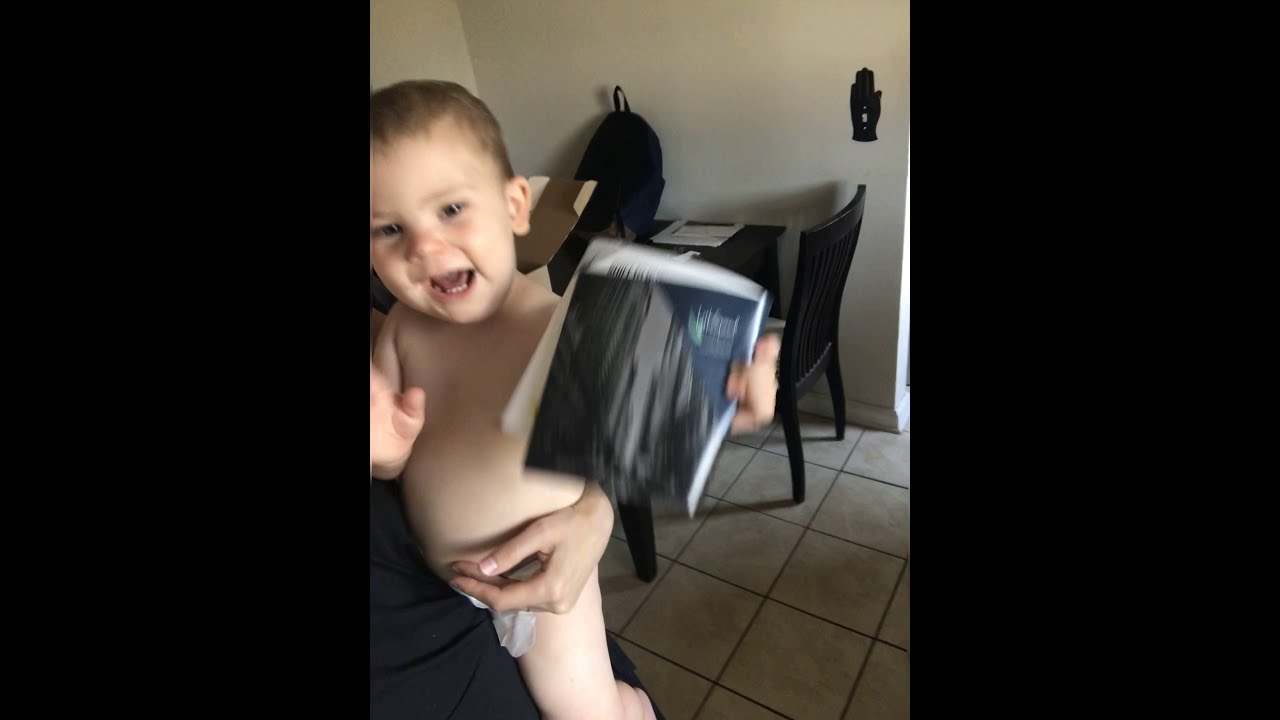The photograph in question is a triptych with two side panels in black and a central photographic image featuring a baby, possibly an infant around two years old, held in the arms of an adult. The baby, dressed only in a diaper, is smiling or laughing with an open mouth, holding a piece of paper or a pamphlet in its right hand, held up towards the camera. The adult holding the baby is only partially visible, with a black shirt and an arm wrapped around the baby’s waist. The background reveals an off-white wall with a light switch and the silhouette of a black hand, a dining table with two chairs, a black backpack on the table, and scattered papers. The floor beneath them is a white and gray textured tile that appears slightly dirty. The lighting in the image seems to emanate from the upper right corner, casting soft light over the scene.